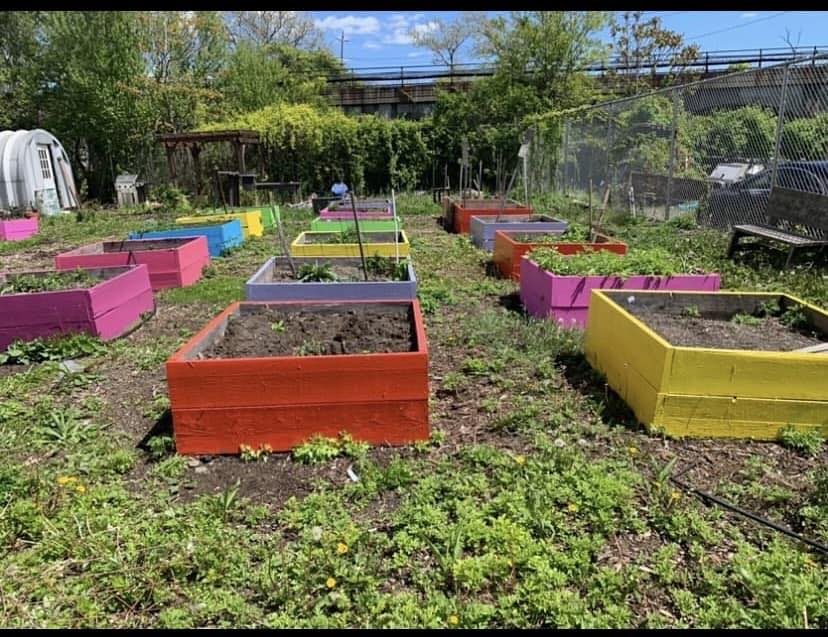The image captures a large square picture taken outdoors, likely in a backyard or nursery, during the daytime with a blue sky and a few scattered white clouds. Dominating the right side of the image is a tall wire chain-link fence, and just beyond the fence, a parked car is visible. Above the fence and stretching horizontally across the image is an older-looking bridge with streaks of brown and a railing.

The foreground and midground are filled with a lush green area dotted with weeds and dandelions, suggesting a backyard setting. Central to the image are three distinct rows of square planters, each row comprising around 6 individually painted planters in a variety of colors including pink, dark pink, blue, yellow, orange, green, and red. These planters are filled with soil, and while most appear to be bare, a few exhibit small green plants or have wooden stakes indicating future planting activity. These vibrant, multicolored planters contribute to a sense of an organized yet casual garden space, possibly part of a community gardening project.